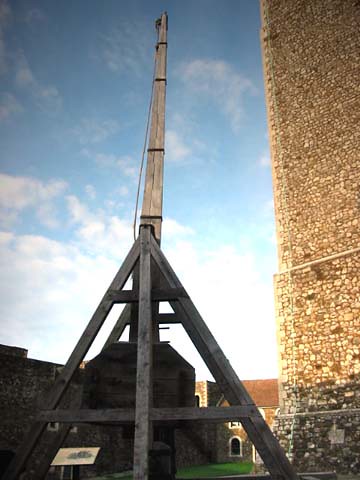In this detailed image, we see a historical village under a partly cloudy, bright blue sky. Dominating the right side of the image is a tall, stone tower made of white and medium stones arranged in a light fashion, extending beyond the top of the photo frame. Adjacent to it, on the left side, stands a unique wooden structure, dark gray in color, resembling a crane or a teepee with three vertical posts connected by crossbeams and capped with a vertical beam. This wooden structure isn't an enclosed building but appears to protect or house a dark, possibly metallic object. In front of this structure, there is a plaque on a small, white podium, likely detailing the historical significance of the site. Surrounding these main features are more cobblestone buildings, including cottage-style houses with visible windows and doors, underscoring the village's historical context.